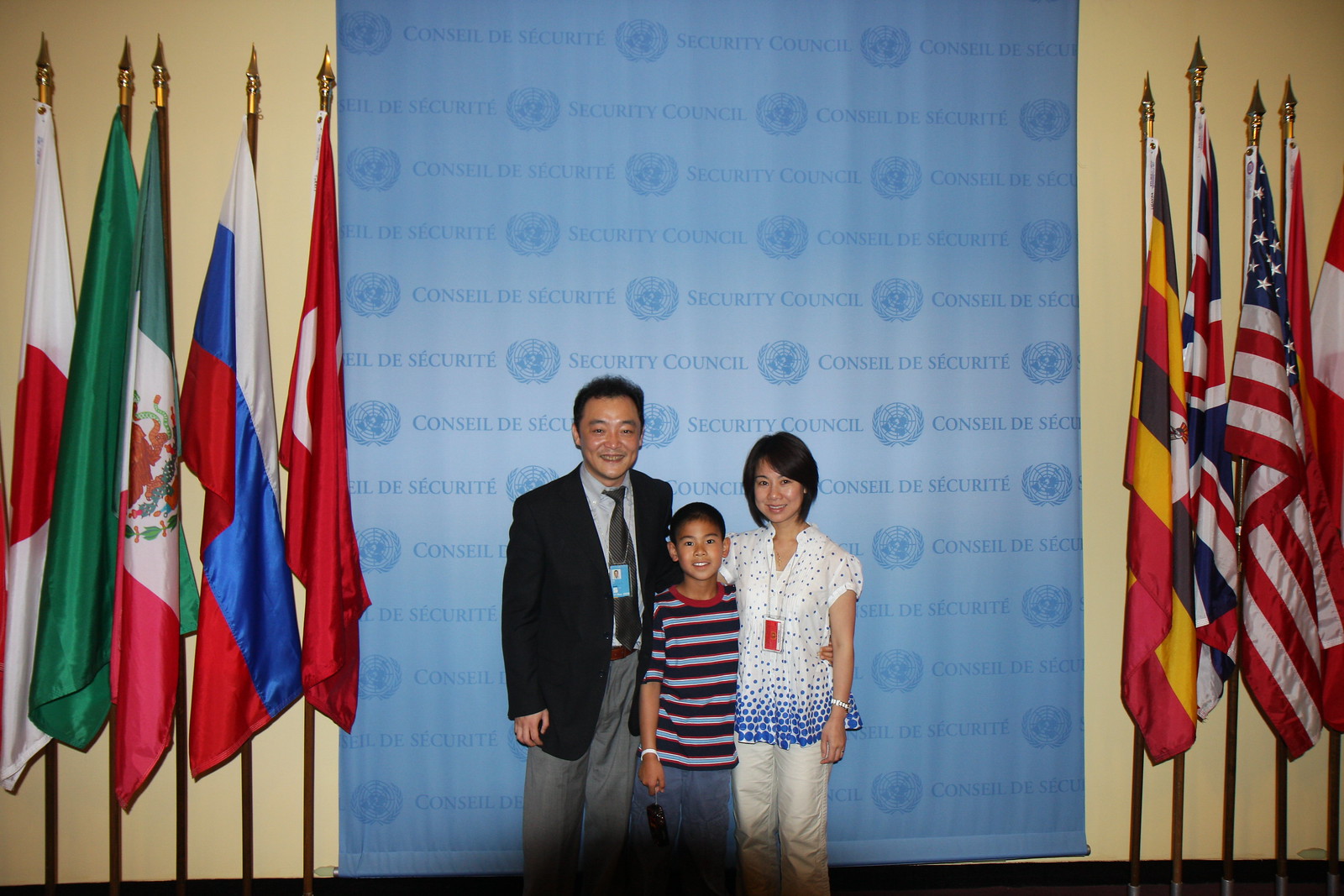The photograph features a family of three, who appear to be of Asian descent, standing in front of a wall labeled "Security Council" with multiple flags in the background. The father, positioned on the left, is wearing a black suit jacket paired with a dark grey tie, a gray button-down collared shirt, gray slacks, and a brown belt, and he has an identification lanyard around his neck. In the middle is a young boy, approximately 10 years old, dressed in a black, red, blue, and white striped shirt with denim jeans, holding an object in his right hand. To the right, the mother is wearing a white blouse with blue polka dots and light-colored pants. They all have short brown hair. The scene is set against a backdrop with five flags to the left and five to the right, including recognizable national flags such as those of Japan, Mexico, the United States, the United Kingdom, Canada, and Germany. The context suggests they might be at a government or international organization building, possibly for an official or celebratory occasion like a citizenship event.